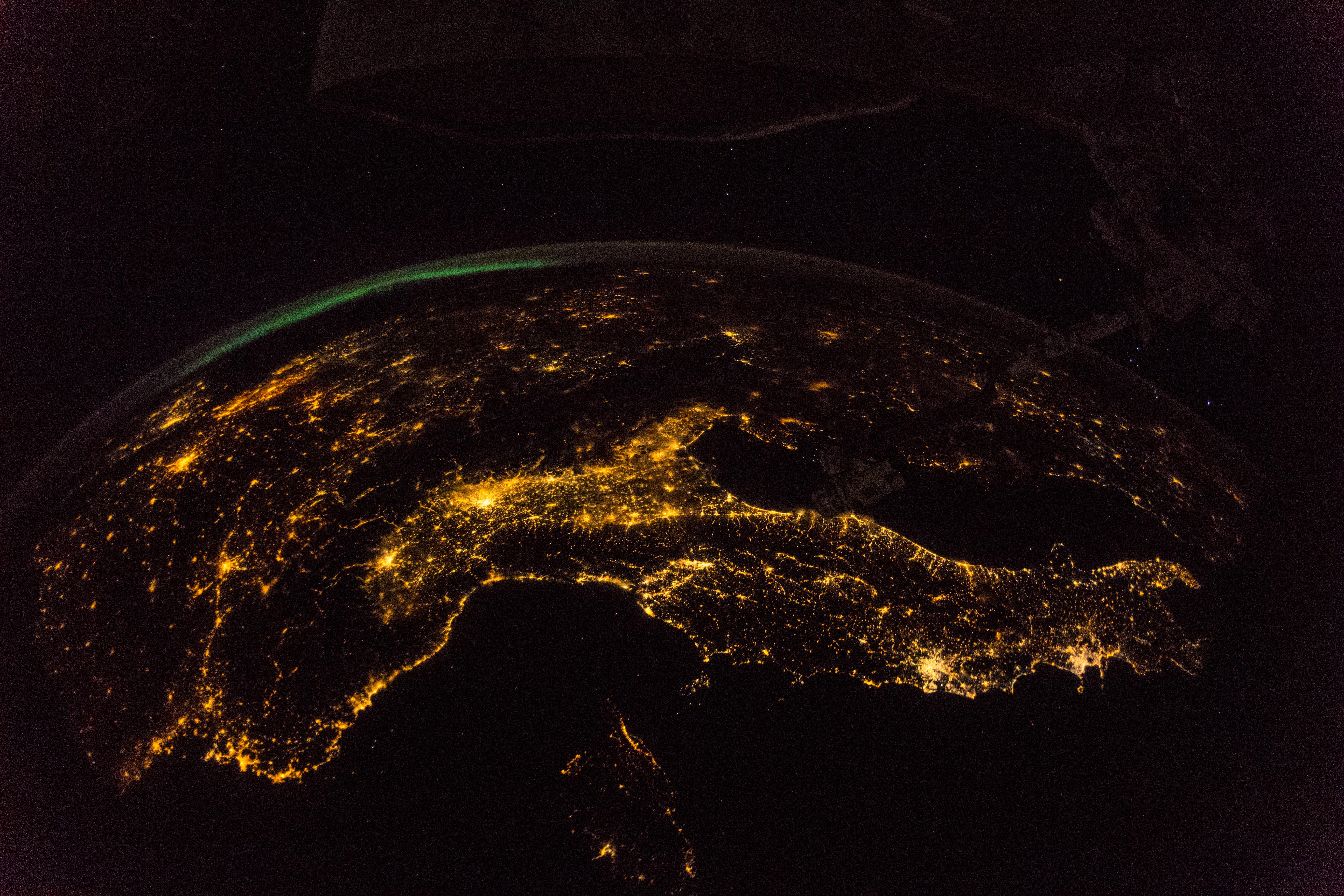This detailed satellite photo of Earth captures a stunning view from outer space, showcasing vibrant city lights scattered across the planet's surface. Prominent is the Italian Peninsula situated in the center-right at the bottom of the image, bordered by the Adriatic Sea to the east and the Tyrrhenian Sea to the west, leading into the wider Mediterranean Sea. The concentrated, bright glows of cities across Italy and other regions create striking yellow hues outlining the continents against the surrounding dark oceans and landmasses. In the upper part of the image, faint green glows suggest the presence of the northern lights, while the background space is a deep black, punctuated by tiny, distant stars. A satellite or space object is visible in the top right corner, adding to the celestial context of the photograph.